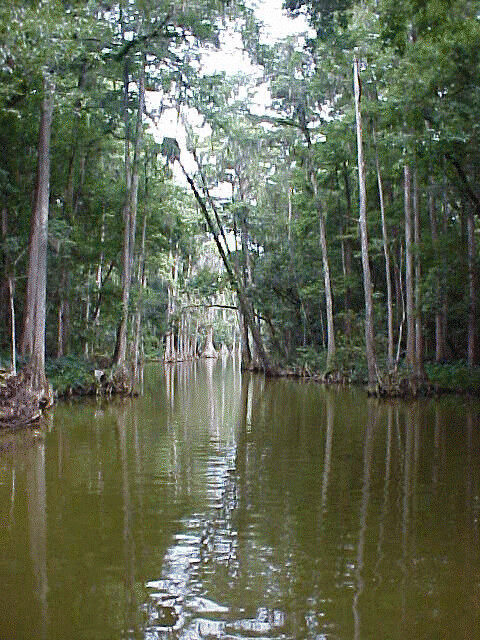The image captures a serene river winding through a marshland. The murky, greenish water occupies the lower portion of the frame, extending into the distance where it curves to the right, giving the scene a captivating depth. On both sides of the river, tall trees line the banks with grassy shrubs and fern-like plants at their bases, creating a rich tapestry of greenery. The sky, barely visible through the tree canopy, appears white and cloudy. A few trees on the right bank bend towards the left, adding a dynamic element to the otherwise tranquil setting. The surface of the water features a couple of ripples, reflecting the sunlight and the silhouettes of the trees, enhancing the overall natural beauty of the scene.